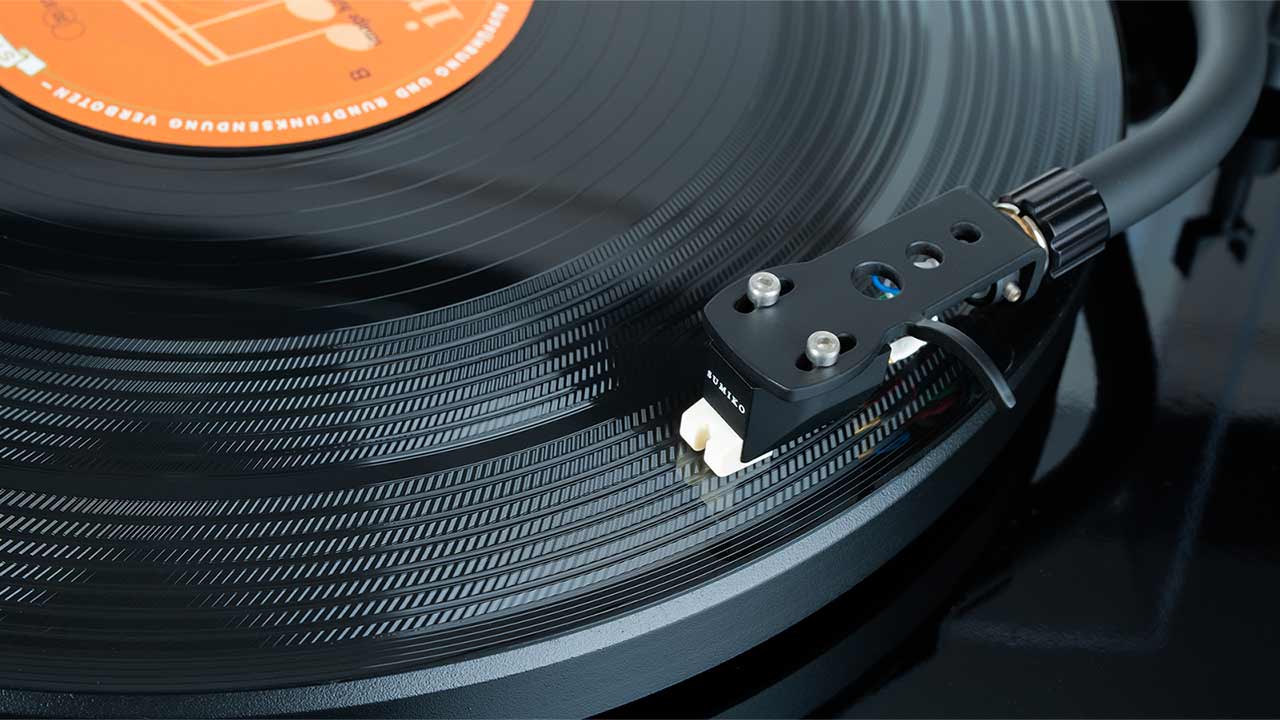The image is a close-up of a black vinyl record being played on a turntable. The focus is on the needle, which is delicately placed on the record. The needle assembly features a black head with a white part that holds the stylus. The text "Sumiko" is visible in white on the side of the head, indicating the brand. The arm of the needle curves gently as it approaches the record, emphasizing its fragile nature. The vinyl record itself is typical black with visible grooves and has an orange label at the center. However, the text on the label is not readable from this angle and distance. The background is dark, enhancing the focus on the turntable and the vinyl. The turntable and the mount it sits on are also black, blending seamlessly with the record.